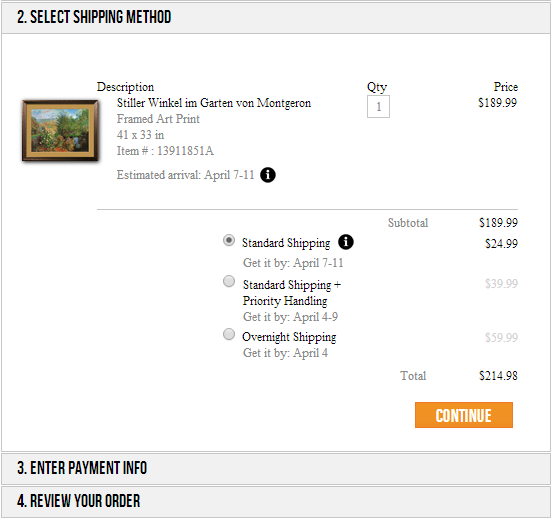A cropped screenshot of a payment screen on an art website is displayed. At the top, a grey banner prominently shows the number "2", indicating the current step: "Select Shipping Method" in bold black text. Below, a thumbnail image of a framed painting is positioned on the left. To the right, detailed information includes the painting's description, title, artist, dimensions, item number, and an estimated arrival date of April 7-11.

In the center of the screen, the quantity is indicated as "1," while the price is listed to the right. A thin black line divides this section from the lower part of the screen, which outlines the shipping costs. The options listed are the subtotal, standard shipping, standard shipping with priority handling, and overnight shipping, with their respective costs displayed on the right. Standard shipping is currently selected.

At the very bottom, future steps in the process are denoted: "3. Enter Payment Info" and "4. Review Your Order."